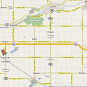This is a small square color image with a beige background, resembling a map. Due to its size, fine details are challenging to discern. The map features several intersecting yellow lines, predominantly vertical, with a thin yellow line running horizontally across the center. In the upper part of the image, slightly left of center, there is a green area, with a smaller green section on the right. Toward the left side, small blue areas are visible. Beneath the thin central yellow line on the left, there is a tiny red object. Centrally from top to bottom, a series of small black marks can be seen, although their exact nature is indiscernible due to the image's diminutive size.